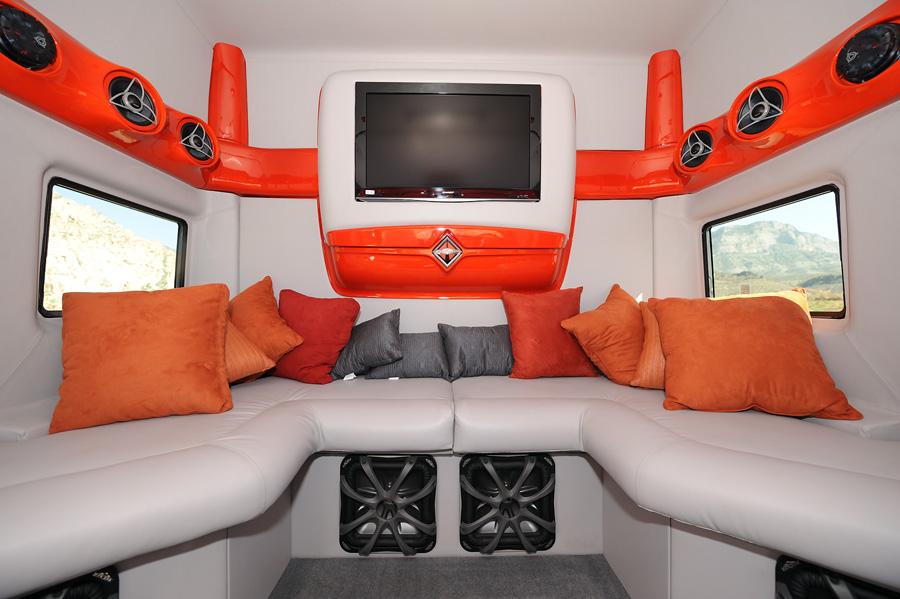This photograph captures the interior of what appears to be a van, RV, or trailer, showcasing a chic and somewhat playful design. Dominating the scene is a white leather sofa, complimented by an array of orange, red, and gray throw pillows, lending a vibrant pop of color. Mounted centrally at the back is a black TV screen that remains switched off, encased in a stylish white and reddish-orange frame. Flanking the TV on both sides are square windows that allow natural daylight to flood in, offering glimpses of an outdoor mountain landscape. Above these windows, an orange band runs around the top, incorporating padded sections near the TV and possibly housing air vents or speakers. Below the sofa, additional vents or subwoofers are visible, contributing to the sleek, seamless aesthetic. The floor is covered in dark gray carpet, which adds to the cozy ambiance of this compact yet sophisticated space.